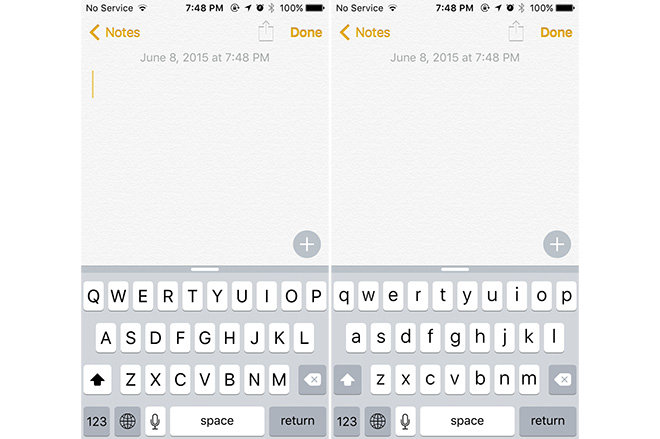This image features an iPhone screen, clearly split into two identical halves, displaying the same content. Both screens show the iPhone battery fully charged at 100% and the time reading 7:48 PM. Despite the active internet connection icon, the status bar indicates 'No Service' with no cellular signal bars visible.

On both halves, the 'Notes' app interface can be seen clearly, with 'Done' button located on the upper right side of the screen. Below the app title, the date and time are displayed as 'June 8th, 2015 at 7:48 PM'. The upper part of the app interface is a blank gray box, devoid of any text or content, creating an empty space on both screens.

In the bottom right corner of each screen, there is a noticeable gray circle featuring a white plus sign in the center. This button is typically used to create a new note within the app. 

Additionally, at the bottom of each iPhone screen, the on-screen keyboard is visible, showing the standard QWERTY layout with letters. In the lower left corner of the keyboard, there is a key labeled '123' which allows users to switch between alphabetical and numerical inputs.

The context, branding, or purpose of this duplicated iPhone screen image remains unclear as there are no business names, promotional clues, or additional imagery provided to explain the specific intent behind this visual representation.